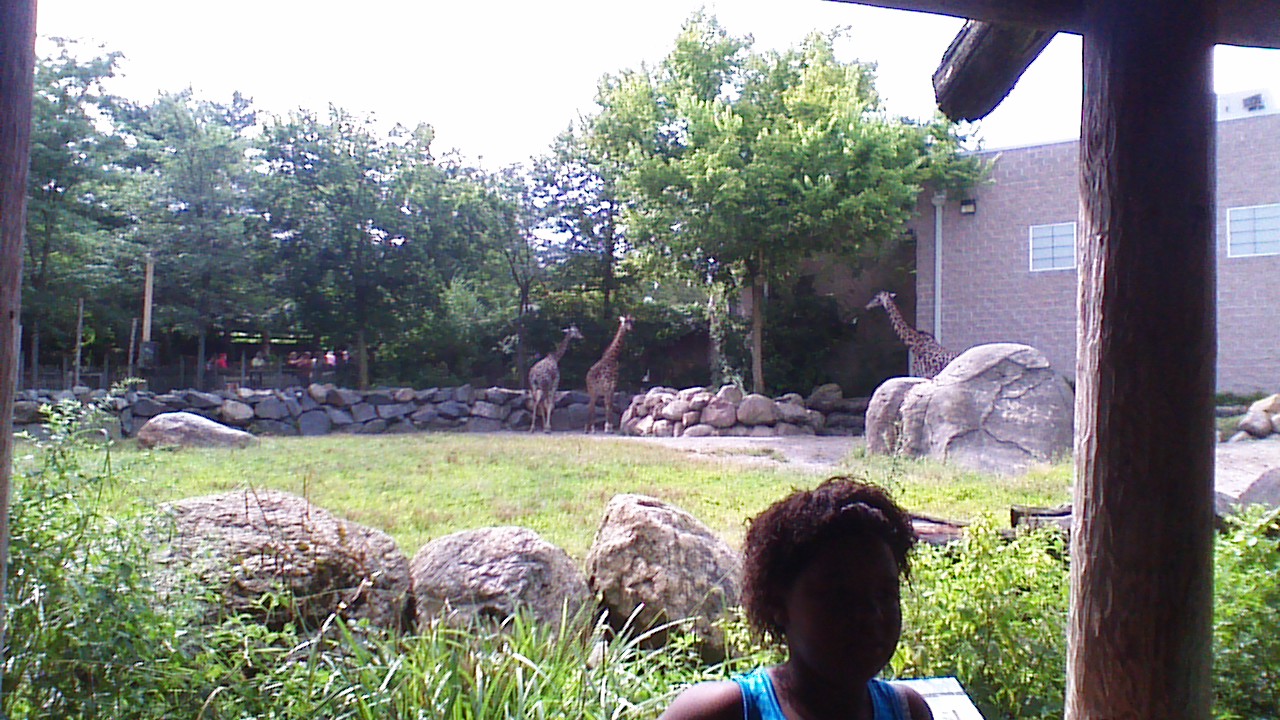This photograph captures an outdoor enclosure at a zoo, primarily focusing on a giraffe exhibit. In the foreground, a young black female with curly hair, dressed in a blue tank top, stands near a large wooden pole, her face obscured by the lighting. The exhibit is lush with green grass, large gray boulders, and various plants. Three giraffes inhabit this space, all positioned away from the camera. A tall tree stands prominently, seemingly dividing the giraffes—two to the left, one to the right. The background features a red brick building with white windows, likely a shelter for the giraffes. Surrounding the enclosure are tall trees and several onlookers standing by a chain-link fence, observing the giraffes. The sky is clear, indicating the photo was taken during daytime.